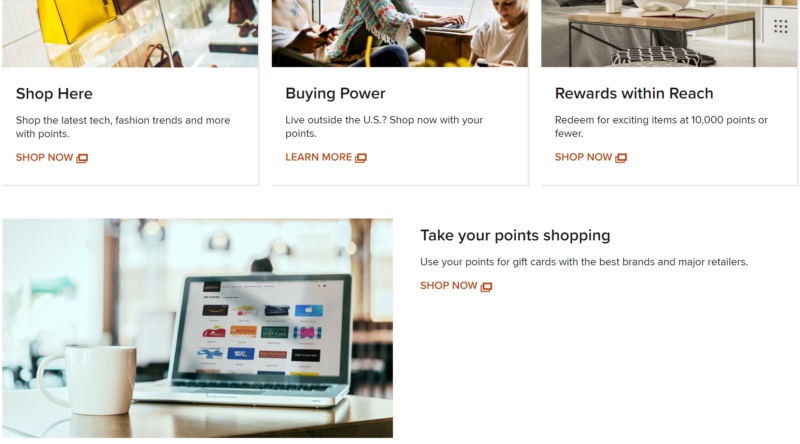A screen capture from a shopping web page, likely related to a points-based rewards system, is displayed. At the top are three rectangular blocks with promotional messages. The first block on the left reads, "Shop Here: Shop the latest tech, fashion trends, and more with points," followed by a "Shop Now" button. The center block states, "Buying Power: Live outside the USA? Shop now with your points," accompanied by a "Learn More" button. The rightmost block declares, "Rewards Within Reach: Redeem for exciting items at 10,000 points or fewer," with another "Shop Now" button below.

Below these blocks, a larger rectangular image is displayed on the left side of the screen, featuring an open laptop on a desk next to a coffee mug. To the right of this image, the text reads, "Take Your Points Shopping: Use your points for gift cards with the best brands and major retailers," along with a "Shop Now" button.

The screen capture lacks company logos or identifying information, and there is no header or footer present on the page. The images and text are colored and structured to guide users towards making purchases with their points, possibly indicating it's a screenshot from a credit card or banking site with a rewards program.